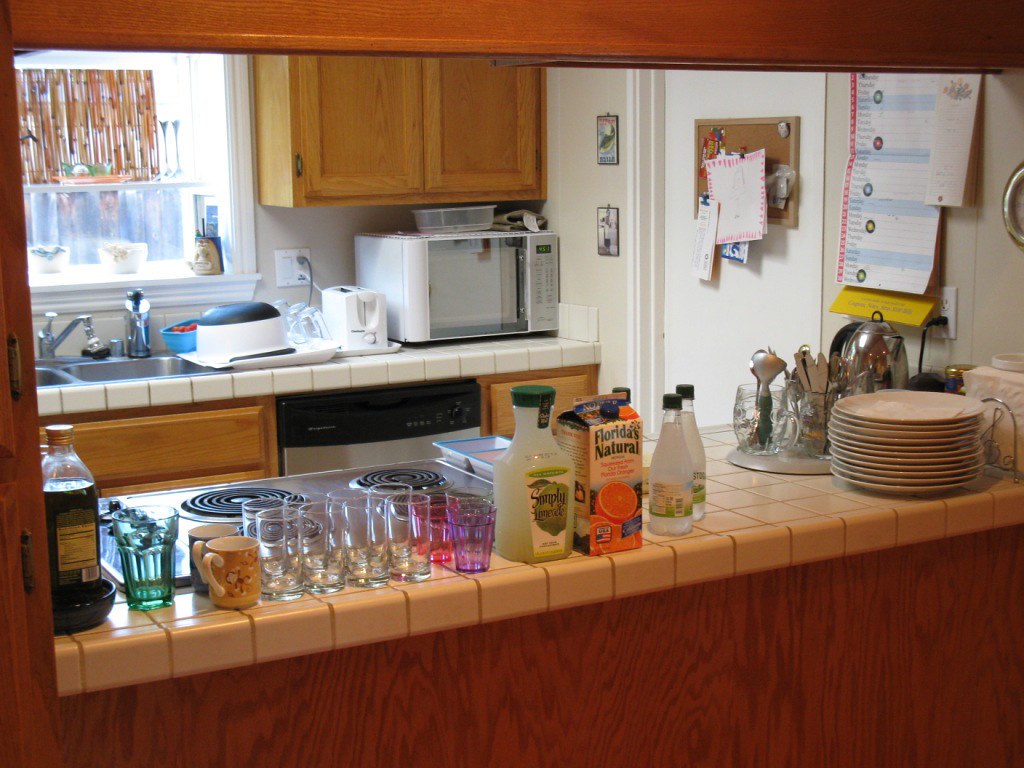This image captures a view from an adjacent room, looking over a bar island into a well-used kitchen space. In the bottom right corner, a distinctly brown wooden surface starts and extends halfway into the image before angling downward towards the left and then stretching upwards off the left edge. This wooden feature is partially overlaid by a countertop that begins just above it, extending further into the frame. 

On the right side of the countertop, a napkin holder accommodates a neat stack of napkins alongside a sizable stack of plates. Positioned behind this arrangement is a tea kettle flanked by two glasses containing unidentified objects. The countertop, with its peach-like hue, showcases an assortment of items towards its edge. Two bottles with green lids precede a box of Florida's Natural orange juice. Adjacent to this, a jug labeled "Simply" in a green label stands. Several glasses, in pink, purple, and clear, are arrayed nearby, accompanied by a brown mug and a blue mug, both adorned with white handles.

To the left of these mugs sits a green glass, which is in close proximity to a cooking oil bottle with a silver top, placed against the brown wooden wall. Behind these items, a silver stovetop is visible, hinting at the kitchen's functional use. Above the array of plates, a wall space hosts various papers, and to the left, a door features a small section for pens and papers. Nearby, two small pictures add a decorative touch to the wall. 

A cabinet occupies the upper left part of the image, with a microwave placed beneath it, resting a plastic bowl on top. Left of the microwave, a white toaster plugs into a wall outlet slightly up and to the right. Adjacent to the toaster, a small strainer holds various dishes. In the top left corner of the image, a window with a white seal sits just to the left of the cabinet, bringing in natural light. Below the strainer, a silver sink is situated, accompanied below by a dishwasher, distinguished by its black top and silver bottom. The image offers a detailed, comprehensive look into a bustling kitchen filled with everyday items.